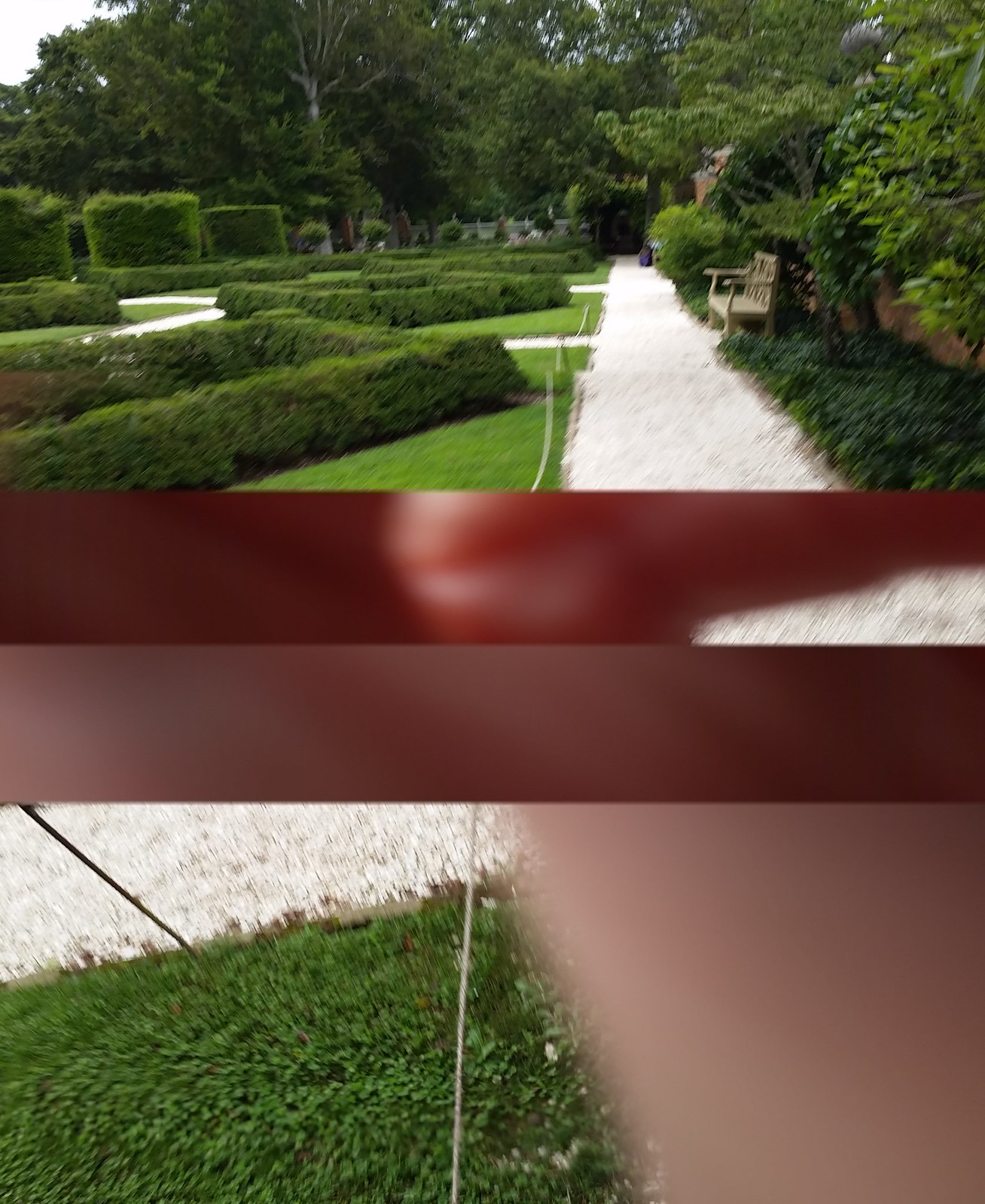The image depicts a meticulously maintained English garden, characterized by its beautifully arranged box-shaped hedges that create a structured and elegant layout. Gravel walkways weave between the hedges, offering a defined path for visitors. Along these pathways, brown wooden benches with armrests provide places to rest and enjoy the serene atmosphere. A striking element in the image is a red, concave support structure that appears to be aiding in the distribution of gravel, indicating ongoing maintenance. Evidence of this work is seen in the scattered gravel along the grass, with a small portion missing in one corner. Additionally, the walkway is partially roped off with small supports, further signifying that upgrades or repairs are in progress.